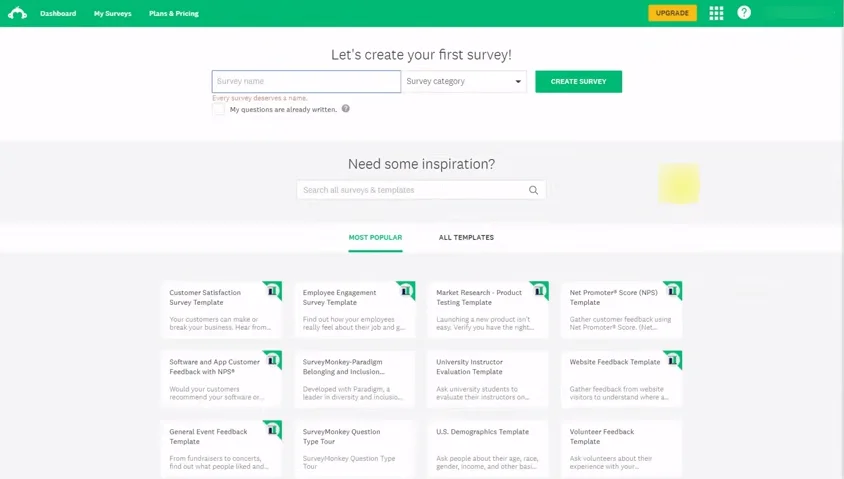The screenshot captures the web interface of the SurveyMonkey website.

In the top-left corner, the SurveyMonkey logo—depicted as a stylized monkey head—is prominently displayed. Just to the right of the logo, a navigation menu features the following options in small white font: Dashboard, My Surveys, and Plans and Pricing. On the far right of the navigation bar, a bright yellow "Upgrade" button is presented, followed by an ellipsis (dots) icon and a question mark icon for additional options and help, respectively.

Centered at the top of the main content section, a bold black heading announces, "Let's Create Your First Survey." Below the heading, a series of interactive elements are aligned horizontally. These include a text box labeled "Name" for entering the survey title, a dropdown menu for selecting the "Survey Category," and a green button labeled "Create Survey" on the far right.

Beneath this setup, another centered heading reads, "Need Some Inspiration?" Directly below this, a search box allows users to find specific templates. Continuing down the page, two categories of templates are presented: "Most Popular" and "All Templates." The "Most Popular" category is currently selected, displaying twelve survey template boxes below, each offering a brief description. Several of these boxes feature a green icon in the corner, indicating that the content requires a paid subscription. 

The overall layout is clean and user-friendly, guiding users through the initial steps of survey creation with intuitive design features.